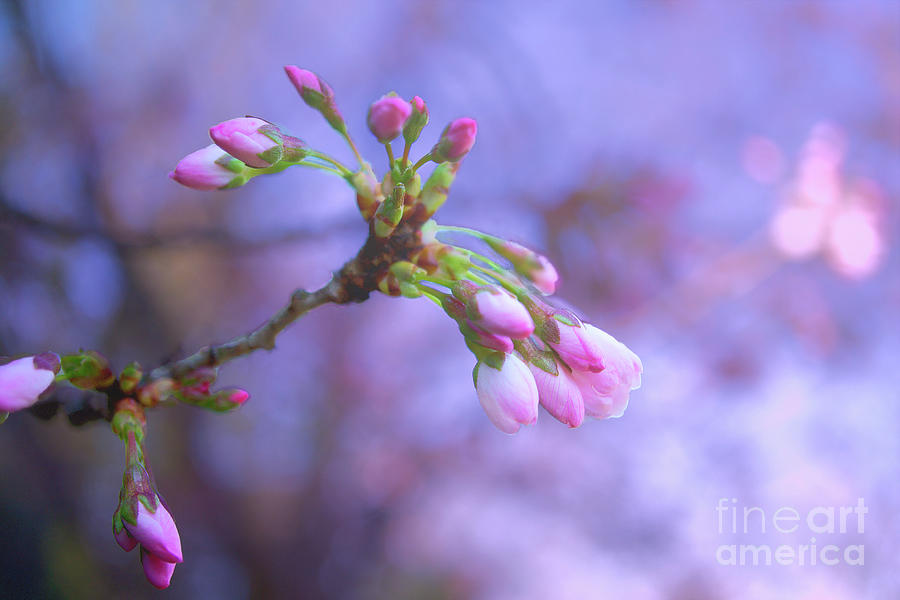This detailed color photograph captures the intricate beauty of a plant on the verge of blooming, possibly a magnolia tree. At the center of the hazy, purply-pink and light blue background, a single green stem extends, adorned with an array of pink flower buds. Counting approximately 13 buds, the flowers are in various stages of opening, ranging from tightly closed dark pink to partially open lighter pink blossoms. The buds grow in clusters along the brownish-gray stem, some even speckled with tiny red tips. The scene is framed by occasional leaves that add a touch of green to the predominantly pink palette. In the lower right corner, white text reads "Fine Art America," subtly marking the photograph.